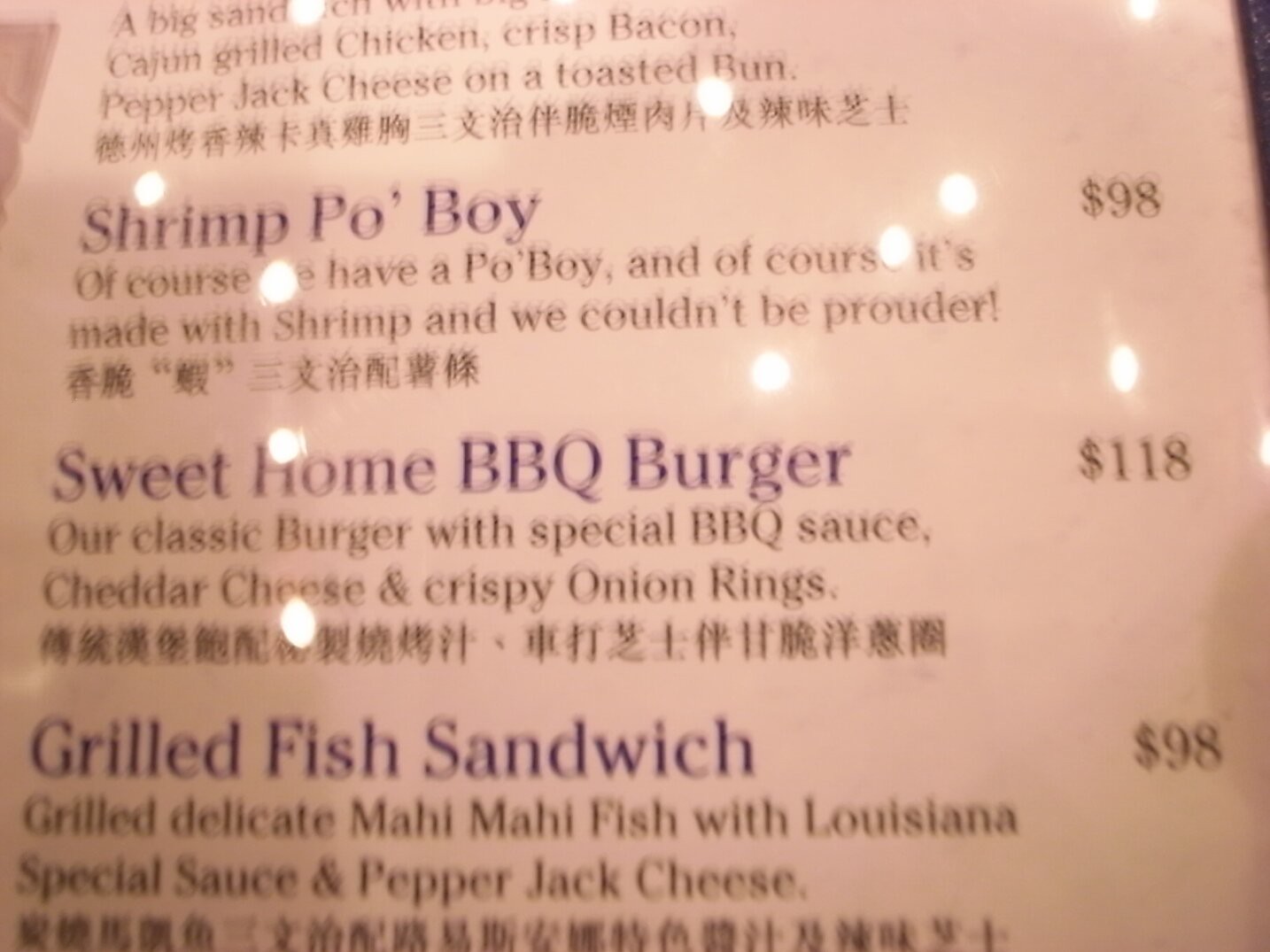The image features a pink menu from a high-end American-Chinese fusion restaurant. The menu is bilingual, with item descriptions in both English and Chinese, reflecting its blend of cultural culinary offerings. Highlighted items include a "Sweet Home Barbecue Burger," described as a classic burger topped with special barbecue sauce, cheddar cheese, and crispy onion rings, priced at an exorbitant $118. Another notable item is a "Grilled Fish Sandwich," featuring delicate mahi-mahi fish seasoned with Louisiana special salt and pepper jack cheese, priced at $98. The menu's pricing suggests either a unique fusion dining experience or a location in a highly touristy area, where the cost of seemingly basic ingredients is significantly marked up. For example, even the onion rings are listed at around $19-$20, emphasizing the overall high price point of the establishment.